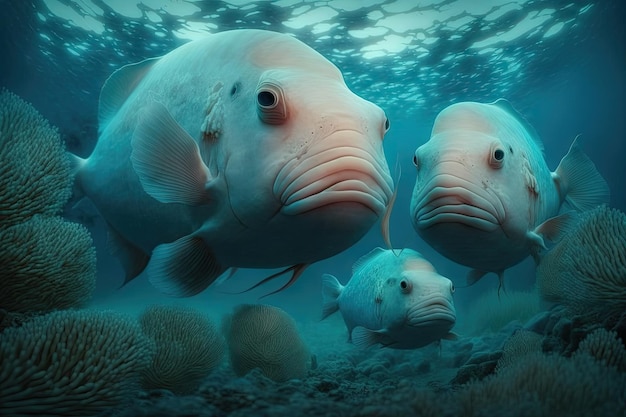In this AI-generated underwater photograph, three large, almost identical fish are depicted swimming amidst a vibrant blue ocean. The fish are a whitish-pinkish hue, with their coloration taking on a slight greenish tint due to the water's glow. They feature wide, big mouths with layered lips and protruding eyes situated on the sides of their heads. The prominent top fin is long and low, while the wide tail fin and the forked fin on their bellies complete their imposing appearance. 

The composition shows the largest fish in the foreground facing slightly to the right, while the second fish, a bit smaller, turns somewhat to the left. The third fish swims at a lower depth in the background, also angled towards the right. Surrounding them, the ocean floor is dotted with various types of coral and rocks. The sunlight filters through the water, creating a pattern of highlights and casting a smooth, almost surreal quality over the scene, accentuating the organized placement of the corals and fish.